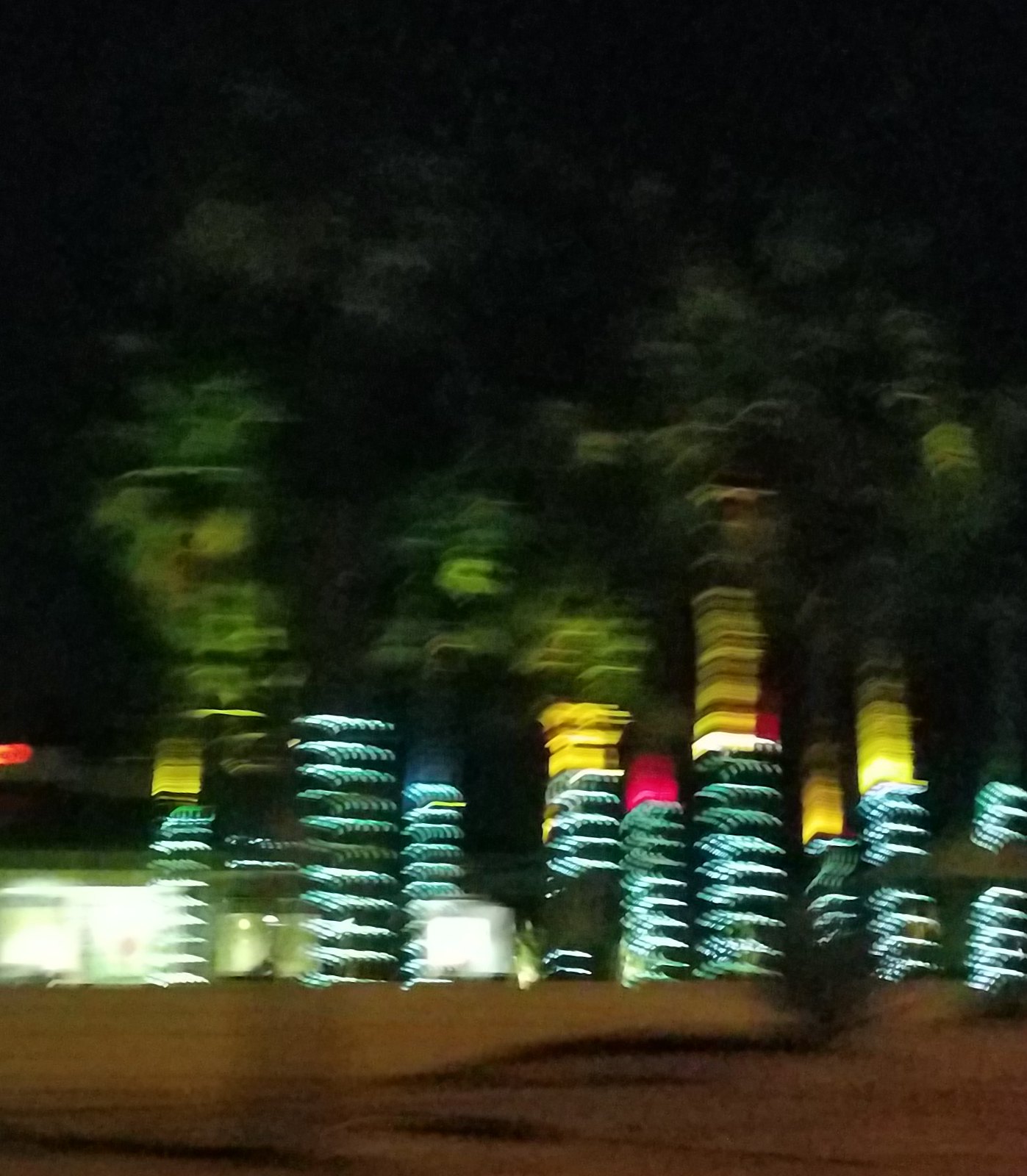This vertical, rectangular image depicts a nighttime scene that is entirely blurred. It showcases a series of poles rising from a wooden base, each adorned with symmetrically arranged lights. These lights, primarily in shades of light blue to white, illuminate the darkness. Some poles extend higher with additional yellowish lights. Topping these structures appears to be foliage, possibly trees or bushes. Toward the bottom left corner of the image, bright lights resembling illuminated windows can be seen in the background, adding to the overall ambiance.